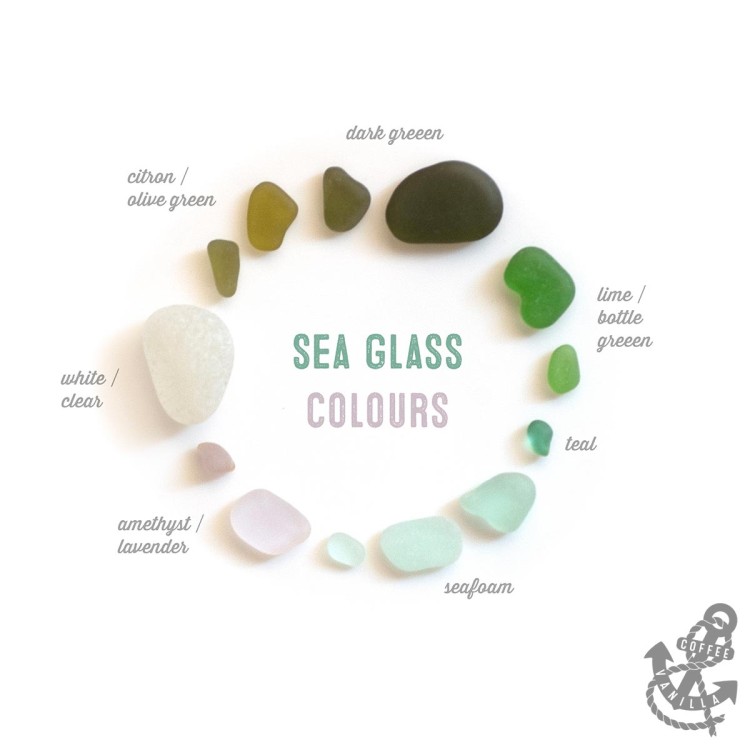This image features an artistic photograph displaying sea glass pieces arranged in a gradient circle on a blank white background. At the center of the circle, the words "Sea Glass Colours" are superimposed in green and gray text. The gradient starts at the top, with dark green stones at the twelve o'clock position. Moving clockwise, these stones transition into lime and bottle green at about three o'clock, followed by teal. By six o'clock, the colors lighten into sea foam, progressing to amethyst and lavender at seven o'clock. Around nine o'clock, the stones are white or clear, and finally, at ten and eleven o'clock, the colors turn into citron and olive green. Each section's color is labeled next to its corresponding stones. The pieces of sea glass vary in size and shape, including small, large, round, oval, and triangular forms. Near the bottom right corner of the image is a logo featuring a gray sea anchor with a piece of rope in the shape of an ampersand, alongside the words "Coffee Vanilla."